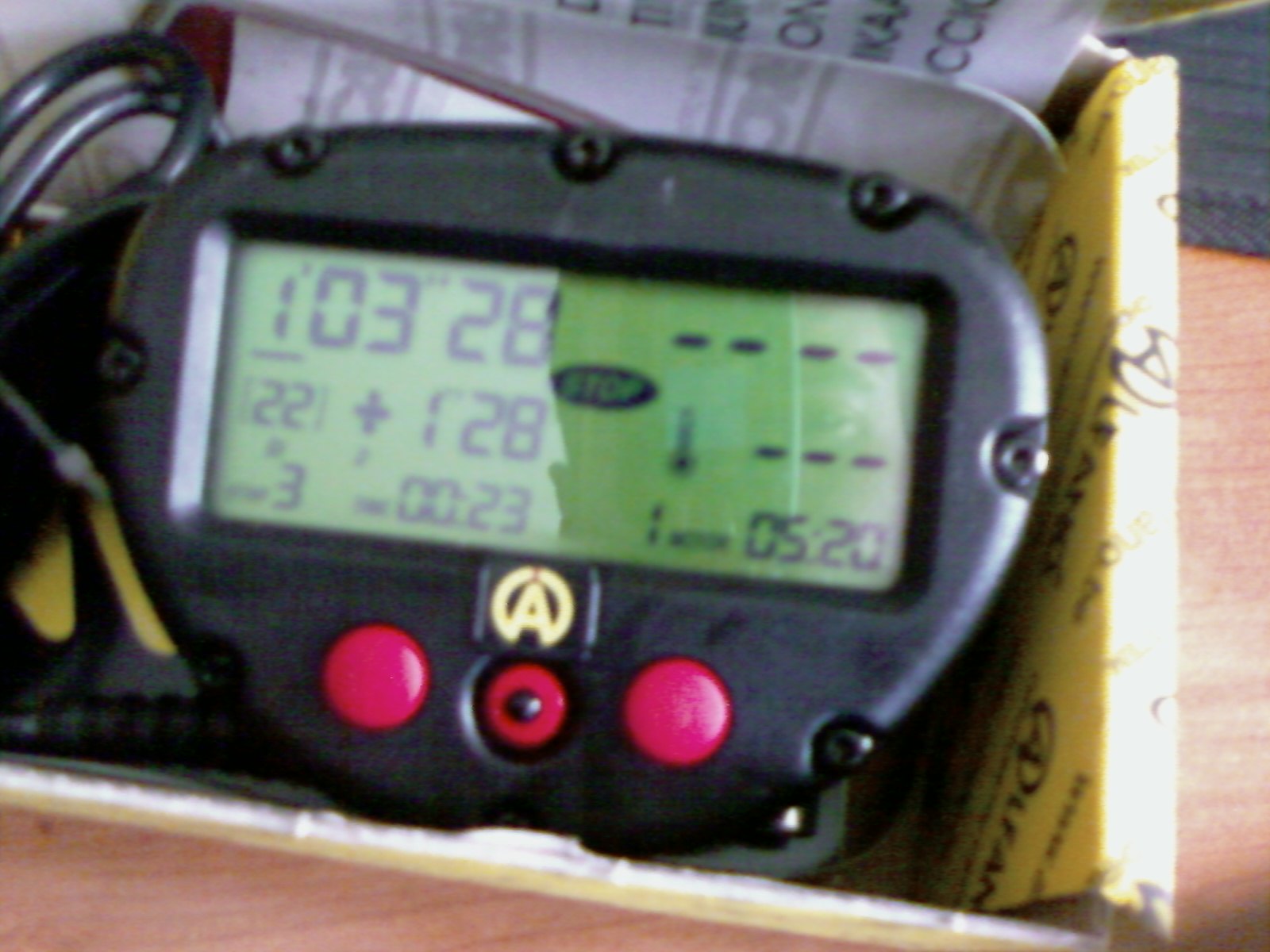The image showcases a detailed photograph of an intricate tool or machine with a slightly rectangular shape that tapers toward the bottom. The device is constructed from black plastic and is secured with tiny screws around its perimeter. It is placed inside a box along with a yellow piece of paper and two white papers. To the left of the main object, a secondary item is visible, zip-tied in place. This secondary object features three red circular buttons at the bottom and a green LCD screen that displays a series of numbers: 1, 03, 28, 22, 3, 05, and 20. The overall setup appears meticulously organized, suggesting a focus on detail and precision.